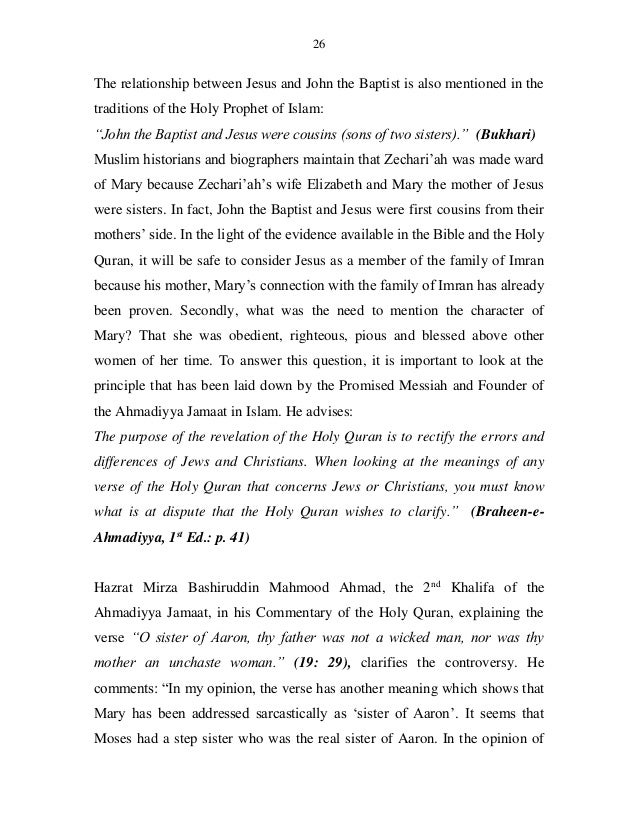The image is a photograph of a written typed page, marked with the number 26 at the top. The page discusses the relationship between Jesus and John the Baptist, as mentioned in both the Bible and the Holy Quran. It details how Jesus and John the Baptist were cousins, the sons of two sisters—Elizabeth, wife of Zechariah, and Mary, the mother of Jesus.

Muslim historians and biographers, including Bukhari, maintain that Zechariah was made the guardian of Mary because of the familial connections. The text asserts that in light of evidence from both the Bible and the Holy Quran, it is safe to consider Jesus as a member of the family of Imran, due to his mother Mary's familial ties. Additionally, the text highlights the character of Mary, emphasizing her obedience, righteousness, piety, and her elevated status among women of her time.

The passage delves into religious interpretations provided by the Promised Messiah and founder of the Ahmadiyya Muslim Community, who posits that the Holy Quran aims to rectify errors and differences between Jewish and Christian traditions. Commentary on the verse “O sister of Aaron, thy father was not a wicked man nor was thy mother an unchaste woman,” is provided, suggesting it addresses historical and religious controversies about Mary. The written text is in black on a white background, and presented in a regular font, with no additional imagery or color.